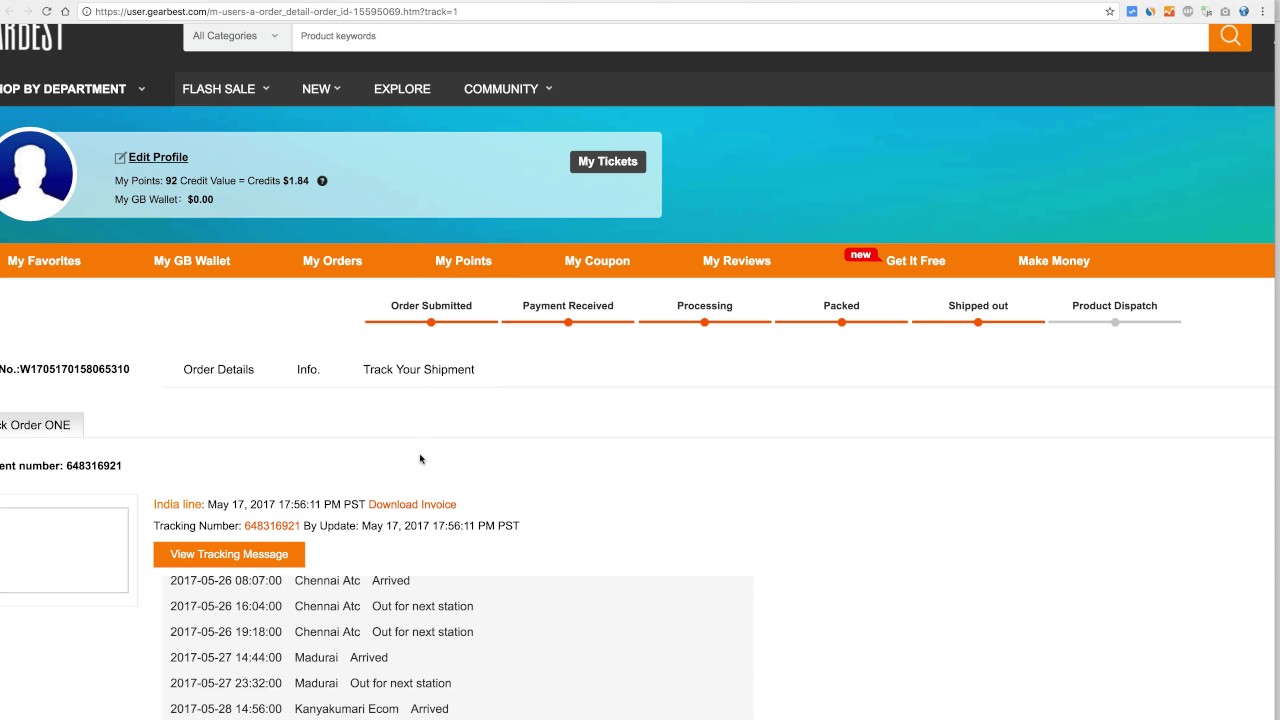The image is a screenshot of a website with a horizontally rectangular layout. At the top, there's a search bar, although the text within it is too tiny to decipher. In the upper left corner, there’s a logo in white font on a black background, but it's partially cut off by the corner, making it unreadable. Adjacent to the logo, "All Categories" is written in gray with a pull-down menu beside it. Following that is a white bar likely labeled "product keywords," and at the far right end of the bar, there’s an orange square featuring a white magnifying glass icon.

Below this, there’s a section with options in white font, although the text is partially obscured on the left edge. It appears to say "Shop by department," with a pull-down menu. To the right of this, on a slightly lighter black background, are the menu options: Flash Sale, New, Explore, and Community.

The next section features a turquoise gradient rectangle that transitions to a more greenish hue toward the lower right corner. On top of this gradient area, a circle is outlined in white but partially cut off on the left edge, displaying a royal blue background with the silhouette of a person in white. Next to the circle, there’s a horizontal, light bluish-green box with "Edit Profile" in black font, which is underlined. Below this text, there are a few lines of text, too small to read clearly. To the right side within a black box, "My Tickets" is written in white.

Further down, an orange rectangle spans the width of the image; it contains "My Favorites" in white font, followed by "My GB Wallet," "My Orders," "My Points," "My Coupon," "My Reviews," and "Get it Free," which has a red flag with "New" in white font attached to it. Lastly, "Make Money" is also listed.

Below this menu is a timeline with steps written in small black font: Order Submitted, Payment Received, Processing, Packed, Shipped Out, and Product Dispatch. Each step has an associated circle below it on a horizontal line. The line under each filled-in step turns orange, except for the final step, Product Dispatch, which remains unfilled.

The subsequent line includes small data points: Order Details, Info, Track Your Shipment. Below this, the detailed order information is provided, though it's too small to decipher. Notably, there's an orange, horizontal rectangular box labeled "View Tracking Message" in white font.